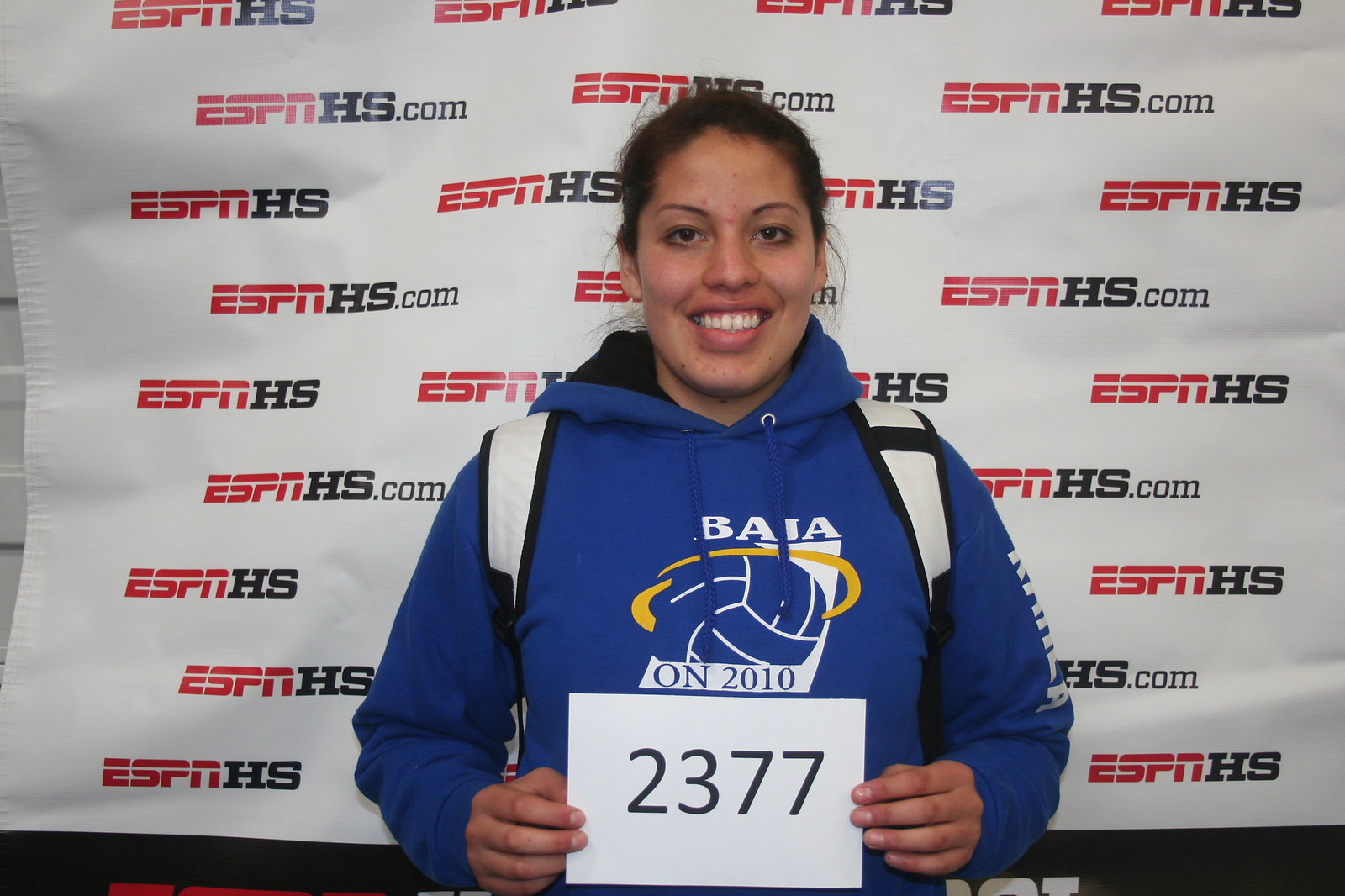In this image, we see a young woman, likely in her 20s, with slightly dark skin and black hair tied back, smiling directly at the camera. She is wearing a dark blue hoodie with a black interior, which features a white soccer ball emblem at the center, and the letters "B.A.I.A." above it. Below the emblem, it reads "ON 2010" in black letters. She carries a backpack, with the white straps visible on her shoulders. Holding a white card with the number "2377" printed in black with both hands, she stands in front of a white plastic banner. This banner has the text "ESPNHS.com" repeatedly printed in red and black letters across it both horizontally and vertically, the "ESPN H.S." section being larger than the ".com." Her dark eyes and friendly smile suggest she is quite comfortable in this setting, which appears to relate to an athletic or sports event.